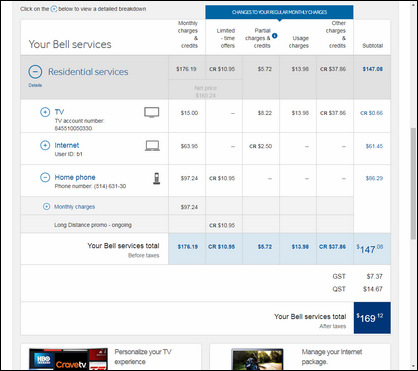Screenshot of a Bell service bill detailing various charges and credits. The header reads "Your Bell Services," followed by a six-column table that categorizes the different billing items. The columns are labeled as follows: "Monthly Charges and Credits," "Limited Time Offers," "Partial Charges and Credits," "Usage Charges," "Other Charges and Credits," and "Subtotal."

In the first column under "Monthly Charges and Credits," several services are listed under "Residential Services," which appears to be a collapsible section. This section contains subheadings for "TV," "Internet," and "Home Phone," each with associated charges. Beside each subheading, there is a collapsible icon, represented by a circle with a minus sign, indicating that further details can be expanded or collapsed.

At the bottom of the table, the bill summarizes the total charges for "Your Bell Services" before taxes. It appears that if there were any business services associated with the account, they would appear in a separate line item above but still contribute to the final total.

The detailed breakdown provides a clear overview of the different services and their respective charges, allowing the user to see both individual and total costs before taxes are added.